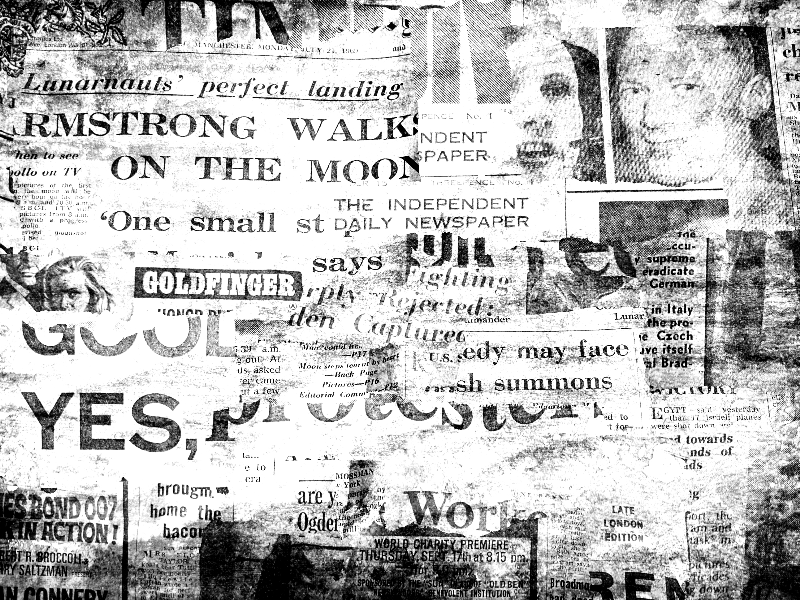This is a detailed black-and-white photo collage composed of classic newspaper clippings from the 1960s, seemingly assembled in a random fashion without a clear organizational pattern. The collage prominently features various headlines, snippets, and images from old-time newspapers. In the upper right corner, there are degraded photographs of a man and a woman, with the woman's face partially overlaid by another newspaper fragment. Dominating the visual narrative, one headline reads "Armstrong Walks on the Moon," with the iconic phrase "one small step" visible underneath, marking the historic event. Additionally, there is an advertisement for the James Bond movie "Goldfinger," displaying the title encased in a black rectangle and showing the faces of Sean Connery and his female co-star. The words "yes" and "Independent Daily Newspaper" are among the many textual elements scattered throughout, alongside other newspaper names like "World, Late London Edition." The collage merges various articles and headlines from that era, creating a nostalgic tapestry that captures a moment in time through its fragmented yet evocative assembly.